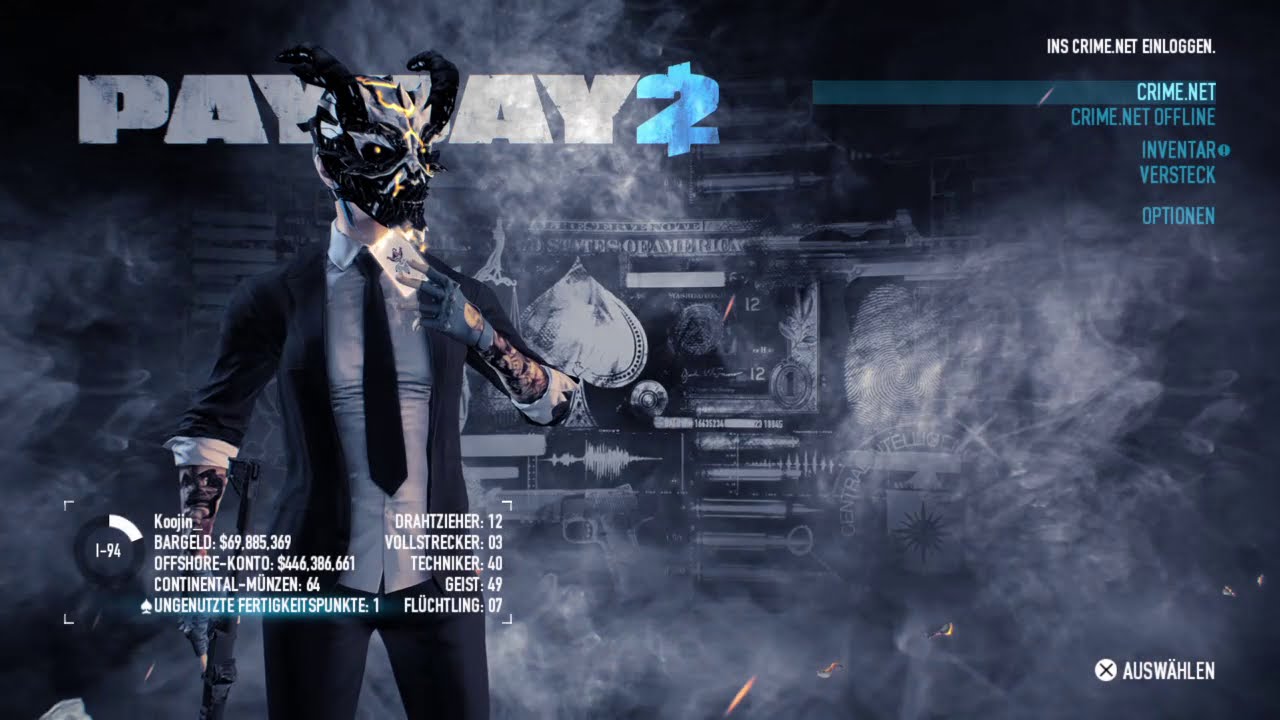The image is a detailed screenshot from the video game **Payday 2**. The scene is enveloped in dark, cloudy smoke that creates an ominous atmosphere. At the center stands a character whose gender is ambiguous, donning a sleek black tuxedo with a long black tie and a white shirt. The character's eerie appearance is accentuated by a black mask with gold electrical bolts and exaggerated alien-like features, including large eyes and a big head. They wear black leather gloves and hold a Joker card up to their face with their left hand, obscuring part of their neck. The right hand, partially covered by overlaying text, appears to be holding a gun pointed towards the ground and sports visible tattoos. 

Surrounding the character are various on-screen elements typical of a video game menu or loading screen. The top left corner prominently features the game's title, **PAYDAY 2**, with "PAYDAY" in white capital letters and "2" in blue, intersected by a vertical line. Additional text and numerical figures, possibly in a foreign language, are scattered across the screen, including leaderboard-like statistics and menu options in the top and bottom right corners. Behind the character, slightly obscured by the smoky ambiance, are graphics resembling a white spade and further textual elements that add to the game’s gritty visual style.